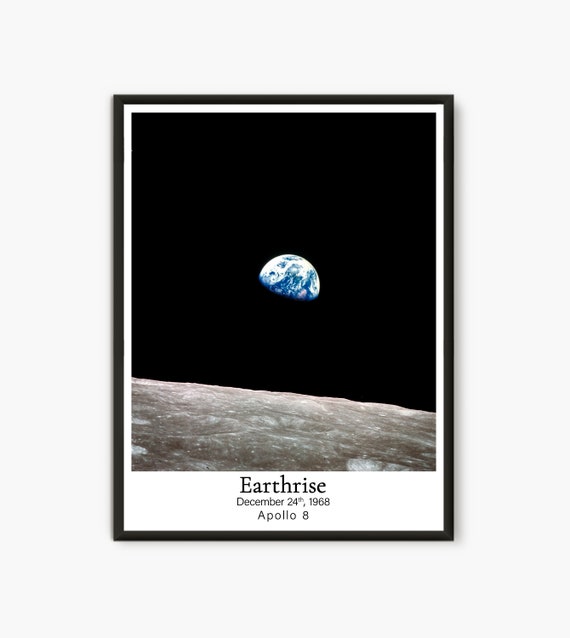The image is a famous photograph titled "Earthrise," taken from the Apollo 8 spacecraft on December 24th, 1968. The image is framed with a black border and displayed on a white wall. The central photograph, which measures approximately three inches high by two inches wide, depicts the Earth partially obscured by the moon's gray, textured surface beneath a stark, black sky. Only the top half of the Earth is visible, showcasing vibrant blue oceans and swirls of white clouds. Below the photograph, in bold black text, are the words "Earthrise," followed by "December 24th, 1968" and "Apollo 8" in smaller print. The overall dimensions of the framed piece are about five inches high and four inches wide, with a light gray background that contrasts with the black frame and black text, emphasizing the significance of this iconic moment in space exploration.